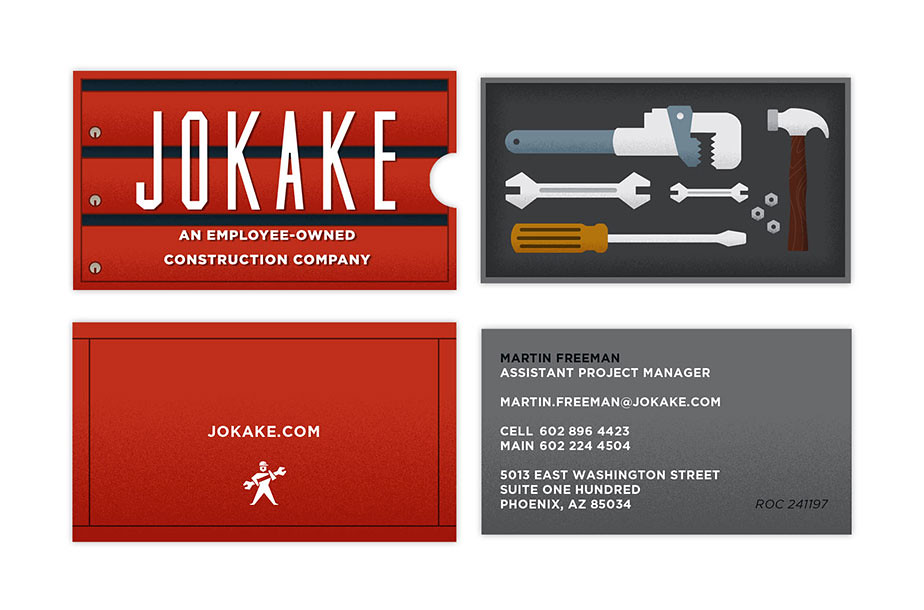This is a four-panel advertisement for a construction company, designed to resemble business cards. The top left panel features a design reminiscent of a license plate or toolbox with a red background and black stripes, adorned with little grey circles on the left side. It prominently displays the company name, "JOKAKE," and the tagline "an employee-owned construction company" in white writing. Adjacent to it, the top right panel showcases a top-down view of a toolbox drawer containing various tools including a hammer, a large wrench, two smaller wrenches, a yellow screwdriver, and three nuts. The bottom left panel retains the red background and reads "jokake.com," accompanied by a cartoon graphic of a man holding an oversized wrench. The bottom right panel, dedicated to contact information, lists the name "Martin Freeman" in black, identifying him as the Assistant Project Manager, along with a cell number, main number, and an address, all set in white text.